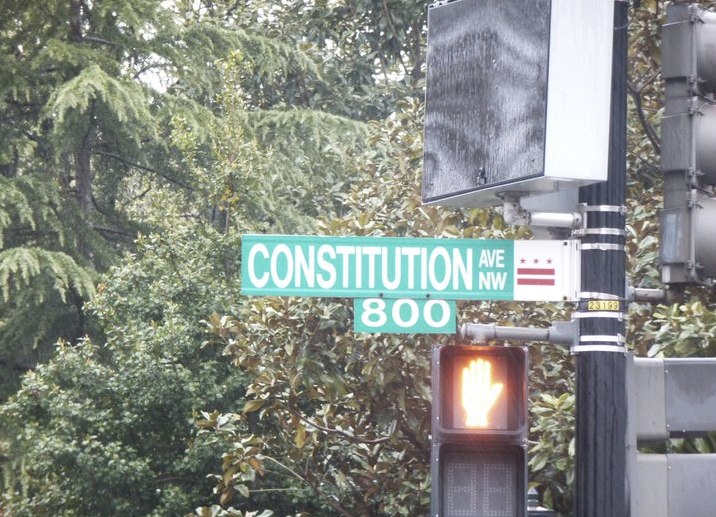The image captures a green street sign with "Constitution" clearly displayed, along with a smaller sign underneath announcing "800." In the background, a cluster of trees provides a verdant, leafy backdrop. Prominently featured in the scene is a pedestrian crossing signal showing a bright red hand, indicating that it is not safe for pedestrians to walk at this time. The juxtaposition of the street sign and pedestrian signal against the lush greenery creates a serene yet urban setting.